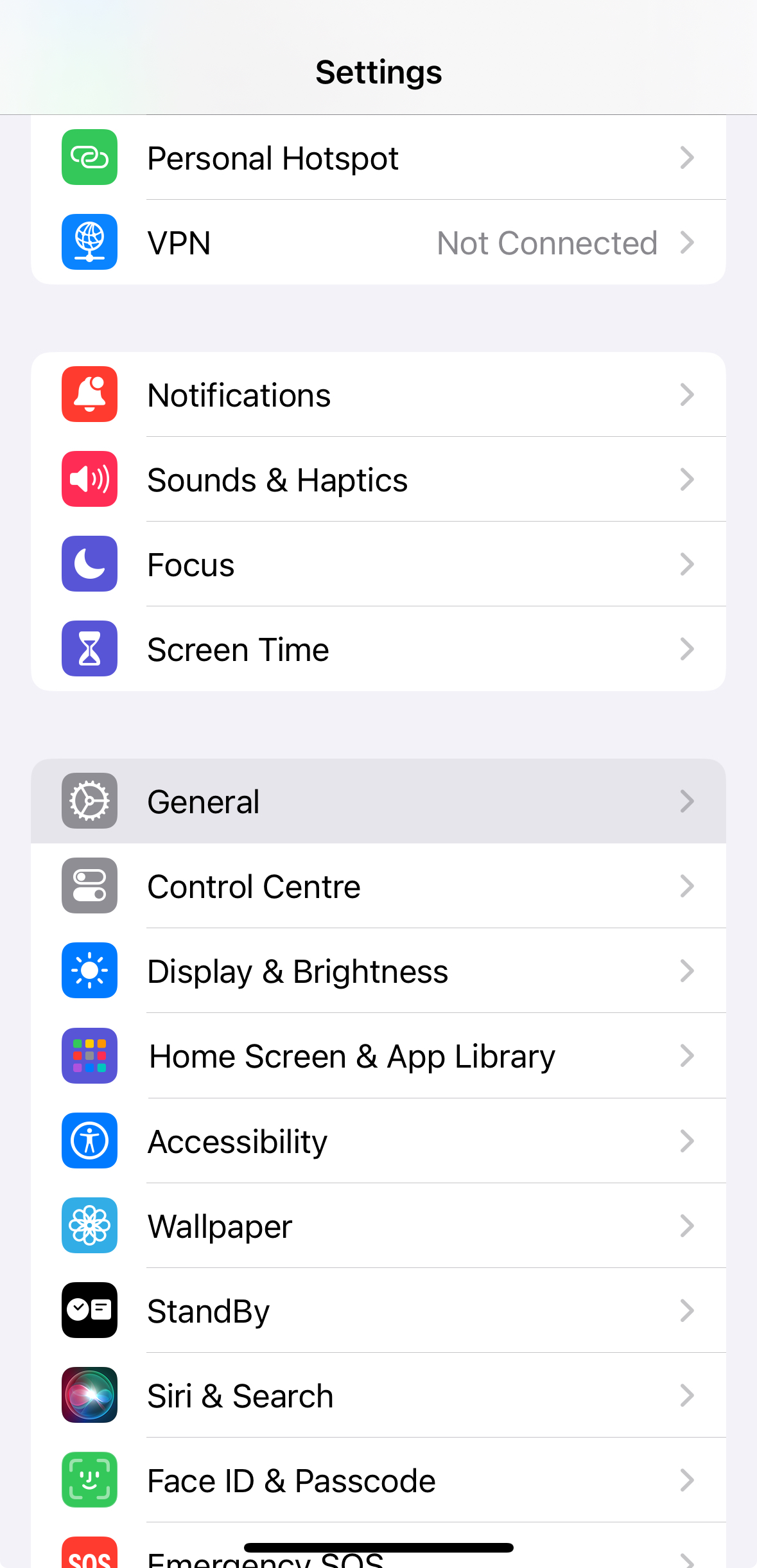The image displays a smartphone settings menu with various configuration options. The background is black, providing a stark contrast that makes the menu items easily readable. Listed vertically, each setting features a right arrow indicating further sub-options. The menu includes:

- **Personal Hotspot** and **VPN**, both marked as not connected.
- **Notifications**, **Sounds & Haptics**, **Focus**, and **Screen Time**, all in white text.
- **General**, notably in gray text compared to the others, indicating it may either be selected or highlighted.
- Additional settings in white text: **Control Center**, **Display & Brightness**, **Home Screen & App Library**, **Accessibility**, **Wallpaper**, **Standby** (stylized as "Standby" with a capital S and B), **Siri & Search**, **Face ID & Passcode**, and **Emergency SOS**.

At the bottom central part of the screen, there is a prominent black bar, possibly for navigation or indicating the current screen view.